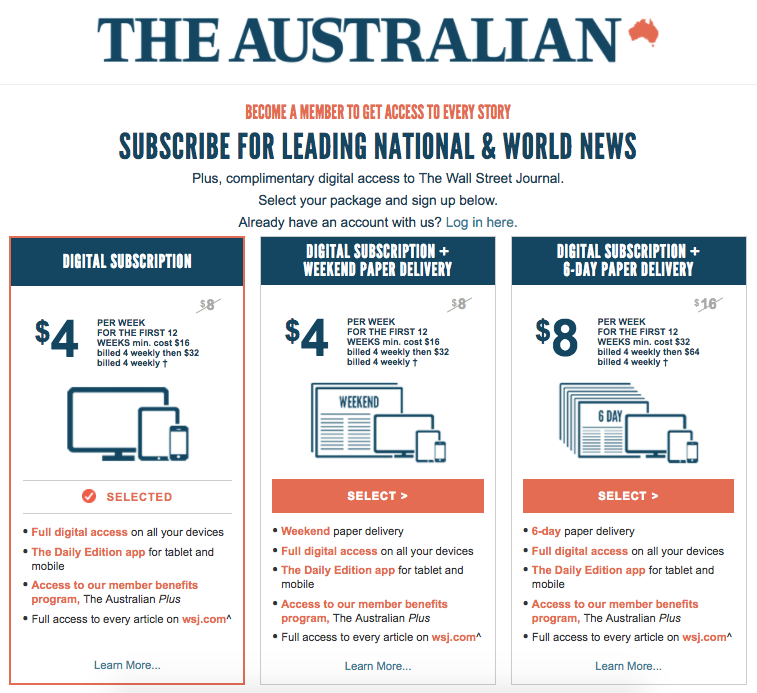A promotional image from "The Australian" magazine features its branding and subscription details. The branding includes "The Australian" written in a dark teal color, accompanied by an orange-coral silhouette of Australia positioned beside the name. Below this, a call-to-action reads in coral: "Become a member to get access to every story." Following this, in teal text, it urges: "Subscribe for leading national and world news," and adds, "plus complimentary digital access to the Wall Street Journal."

Instructions are provided to "Select your package and sign up below." Existing members are prompted with a click-able "Log in here" link. 

The image’s background primarily consists of a white lower section and an upper segment in dark teal, with headings and some sections highlighted in orange coral. Three large rectangles at the bottom present subscription options. The first plan, highlighted and bordered in coral, offers a digital subscription for $4 per week for the first 12 weeks (minimum cost $16), then increases to $32 per four weeks. The other two plans, priced at $4 per week and $8 per week respectively, include "Select" buttons but are not highlighted as selected.

This structured design clearly delineates the choices available to potential subscribers.